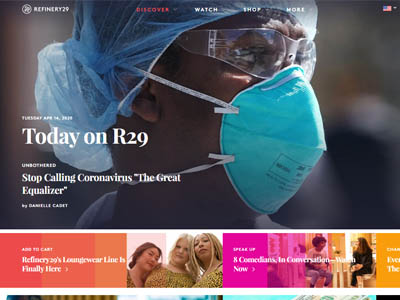This screenshot is from a medical-themed section of the website Refinery 29. At the top left corner, the site's logo "Refinery 29" is displayed in white text. The navigation menu stretches across the top and includes options such as "Discover," "Watch," "Shop," and "Home." On the far right side of the menu, there is a small American flag accompanied by a drop-down button, presumably for language or regional settings.

Dominating the screen, an image occupies about 80% of the space. This image depicts an African-American individual wearing medical protective gear: a blue face mask, goggles, and a blue hairnet. The person is looking off to the right and only their head is visible in the frame. To the left of this individual's head, text reads "Today on R29: Stop Calling Coronavirus the Great Equalizer."

At the bottom part of the screen, two rectangular features are displayed. The first, an orange rectangle, advertises Refinery 29's new Lounge Wear line, showing an image of three women standing next to each other. The second is a pink rectangle promoting an article titled "8 Comedians in Conversation," featuring an image of two people seated at a table.